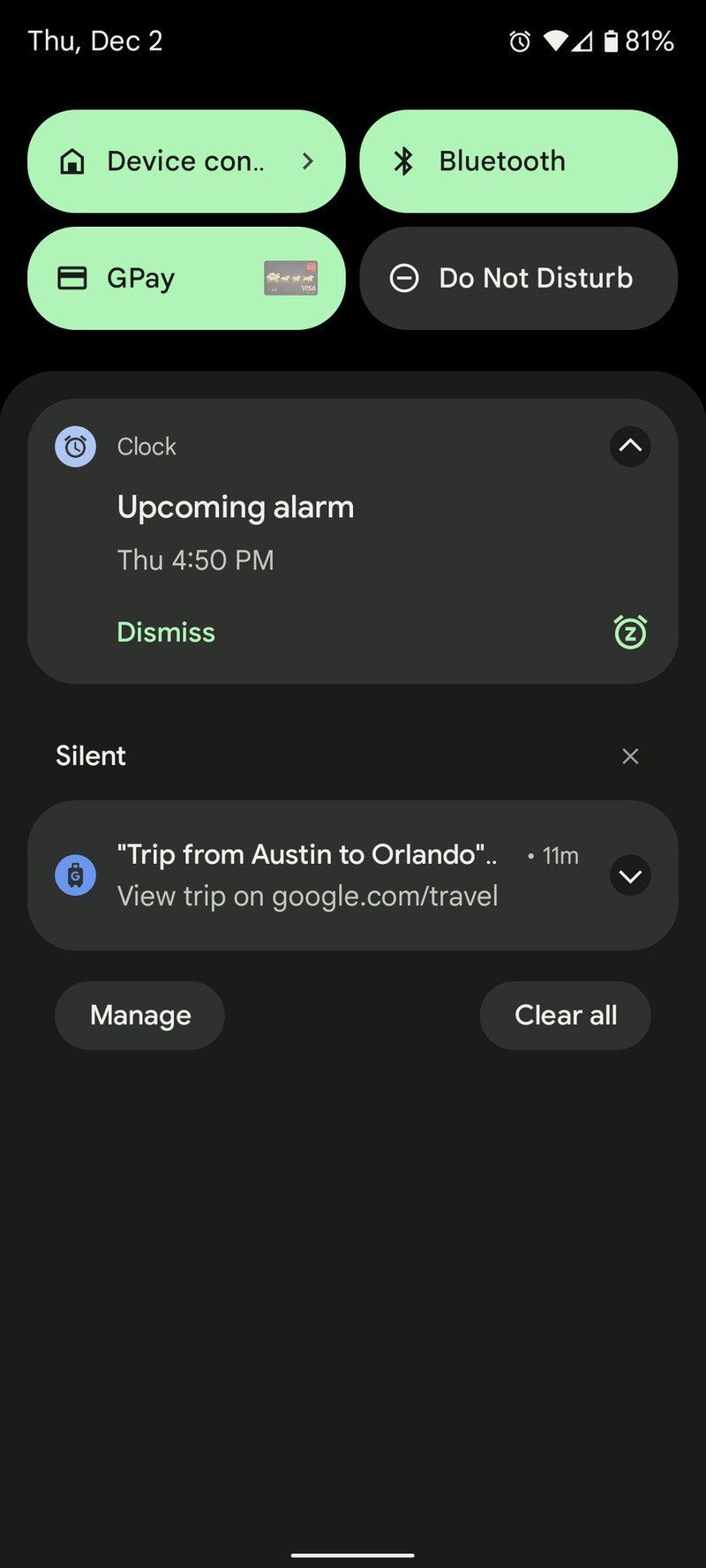The screenshot displays several key details:

**Top Status Bar:**
- **Battery Life:** 81%
- **Date:** Thursday, December 2nd, displayed in the top left corner.

**Notification Icons:**
- **Device Status:** Indicated by a green horizontal oval labeled "CON" with a small house icon next to it.
- **Bluetooth Status:** Indicated by a blue horizontal oval labeled "Bluetooth."

**Notifications:**
- **Payment Notification:** A GPay (Google Pay) icon associated with a credit card image.
- **Do Not Disturb Mode:** Indicated by a horizontal oval labeled "Do Not Disturb."
- **Clock Notification:** Features a small clock icon within a blue circle, labeled "Clock." It shows an upcoming alarm set for Thursday at 4:50 p.m., with an option to dismiss the alarm in green. It also mentions that the device is on "Silent" mode.
- **Travel Notification:** Displays "Trip from Austin to Orlando, 11 minutes" and an option to "View trip on google.com/travel."

**Secondary Control Options:**
- **Manage Notifications:** Displayed in a horizontal oval labeled "Manage."
- **Clear Notifications:** Displayed in a horizontal oval labeled "Clear All."

Each element is neatly organized within its respective section for easy readability and interaction.